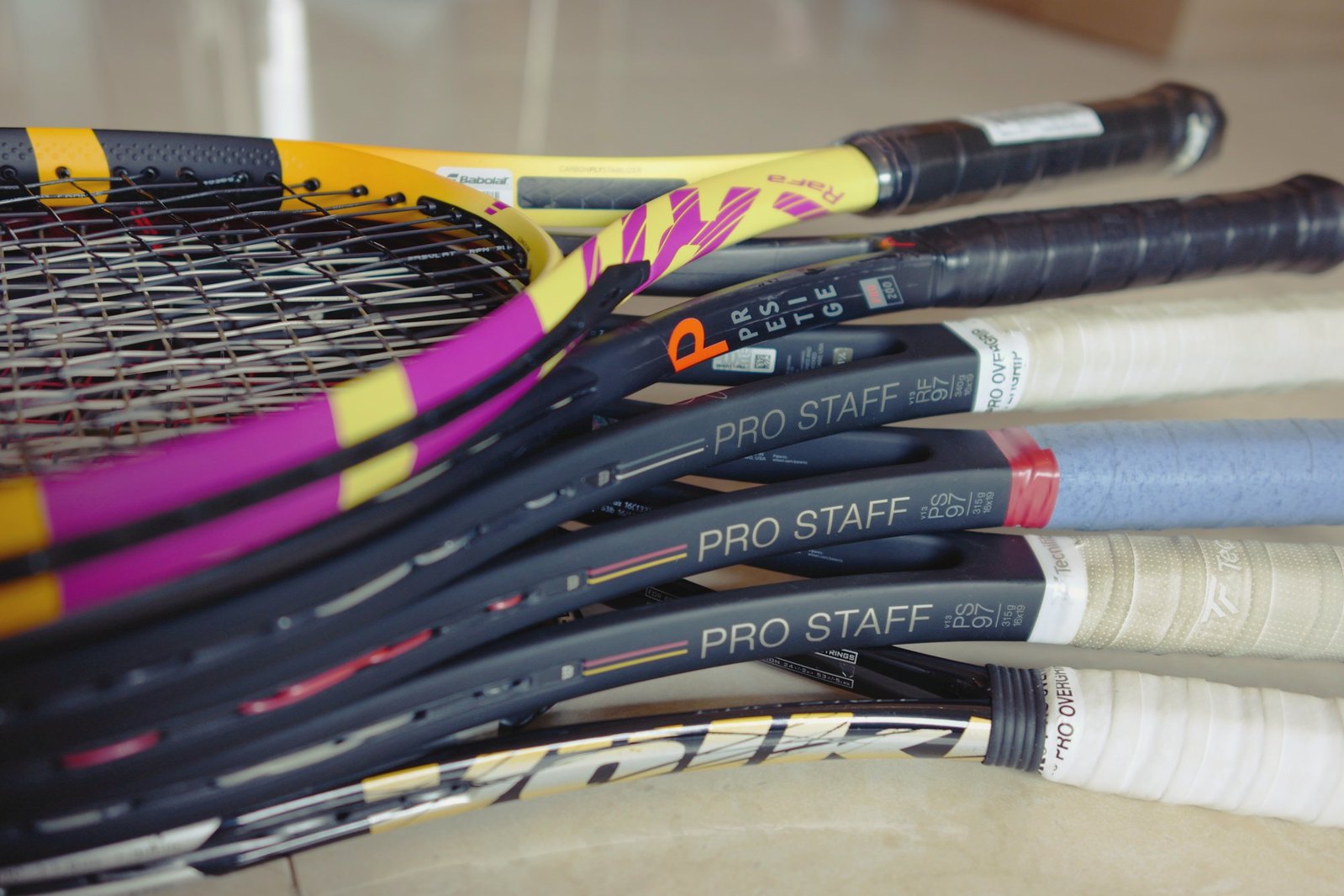The image displays a stack of six tennis rackets viewed from a side profile, laid out on a glossy, beige tile floor that reflects the rackets' details. The rackets are partially cut off at both ends of the image, revealing the variety in handle colors and designs: white at the bottom, followed by blue, another white, and two black handles. The top racket features a yellow and purple design. Just beneath it is a black racket with an orange "P" on the side. The next rackets in the stack, three in a row, are black with "Pro Staff" inscribed in gold font. The racket at the very bottom is black with a large gold bull print that says "Volk". The handles appear slightly turned away from the viewer, creating a subtle fan effect.